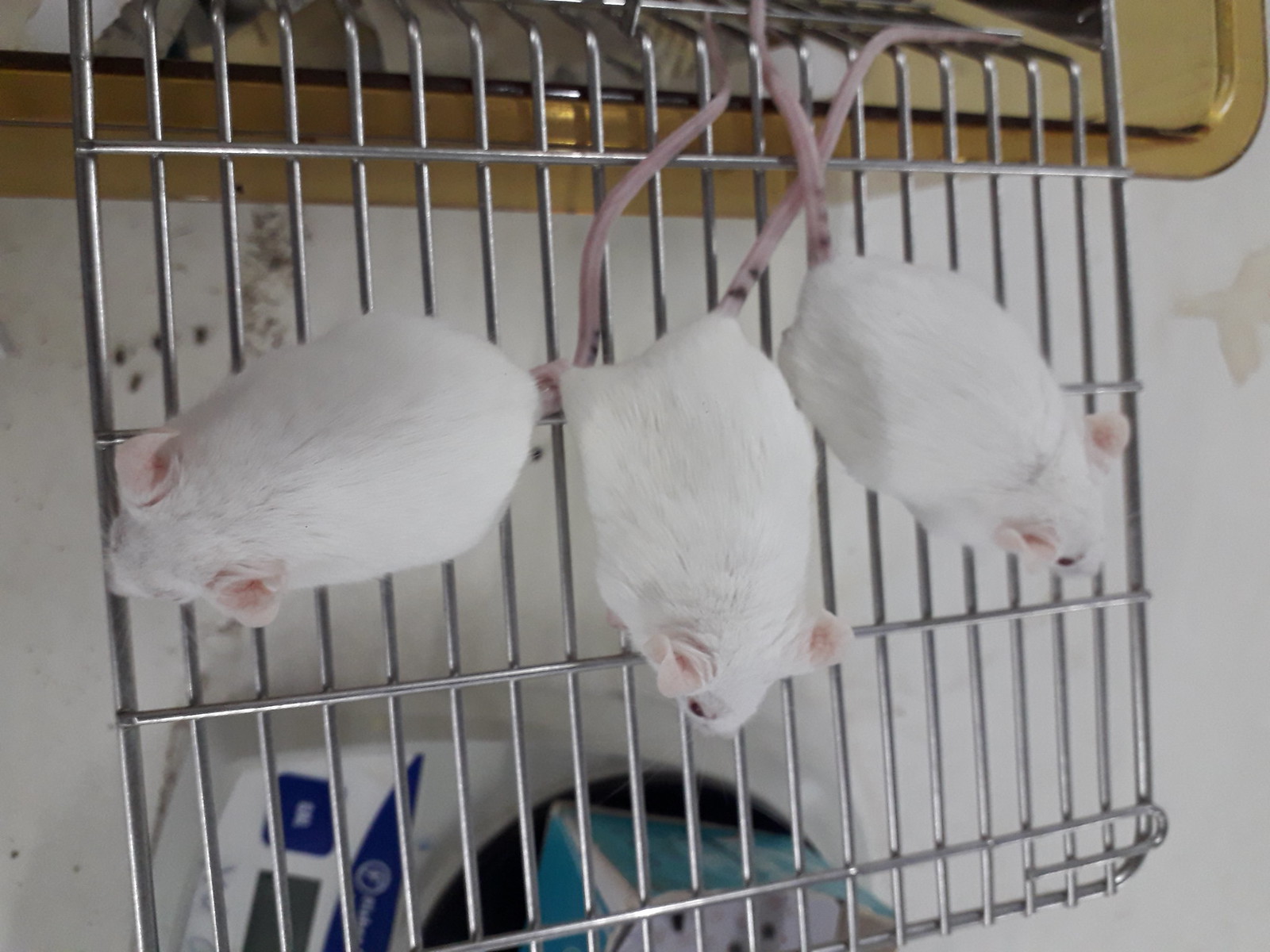In this image, three small, white house mice with pink ears and long pink tails are hanging upside down from a steel rack typically used in sinks to prevent dishes from touching the bottom. The metal rack, featuring a cage-like design with spaces in between, is suspended against a white background. The mice, each about two to three inches long, appear well-fed and content. One mouse is facing left, the second directly downward, and the third to the right, creating a feeling of diverse curiosity among them. Behind them, there is a partially visible sign with gray and blue sections. This detailed perspective is taken from above, emphasizing the unique, playful arrangement of the mice against the clean, white backdrop.